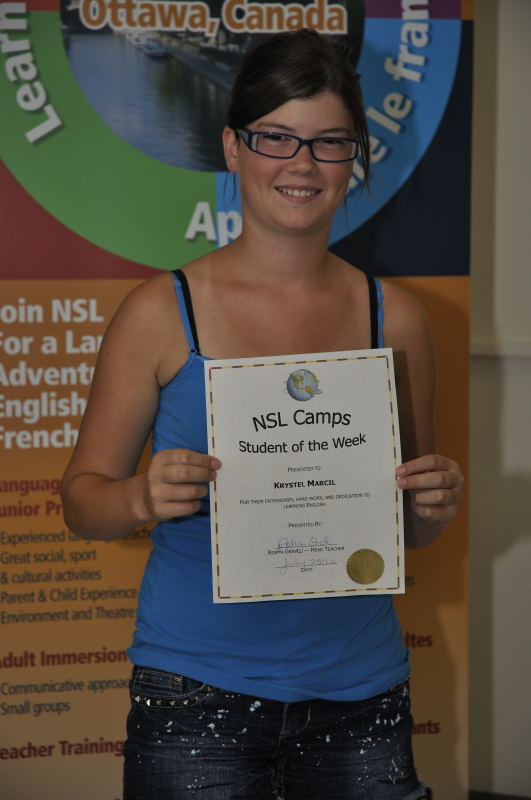This indoor photograph depicts a young woman with short, ear-length black hair and black-rimmed glasses. She is wearing a blue tank top and either black pants or a dark denim skirt. She stands in front of a promotional board that prominently features the words “Ottawa, Canada”, "La France", and “NSL” among other text promoting English and French adventures, although much of it is obscured by her body. The backdrop also includes a mix of colors like green, red, and blue, and possibly an image of a lake. 

In the foreground, the young woman proudly holds up a certificate that reads “NSL Camps Student of the Week, presented to Crystal Marcus,” accompanied by some signatures and a gold medallion or seal in the bottom right corner. The explanatory text under her name is illegible. The award and the beaming smile on Crystal’s face capture a moment of achievement and pride.